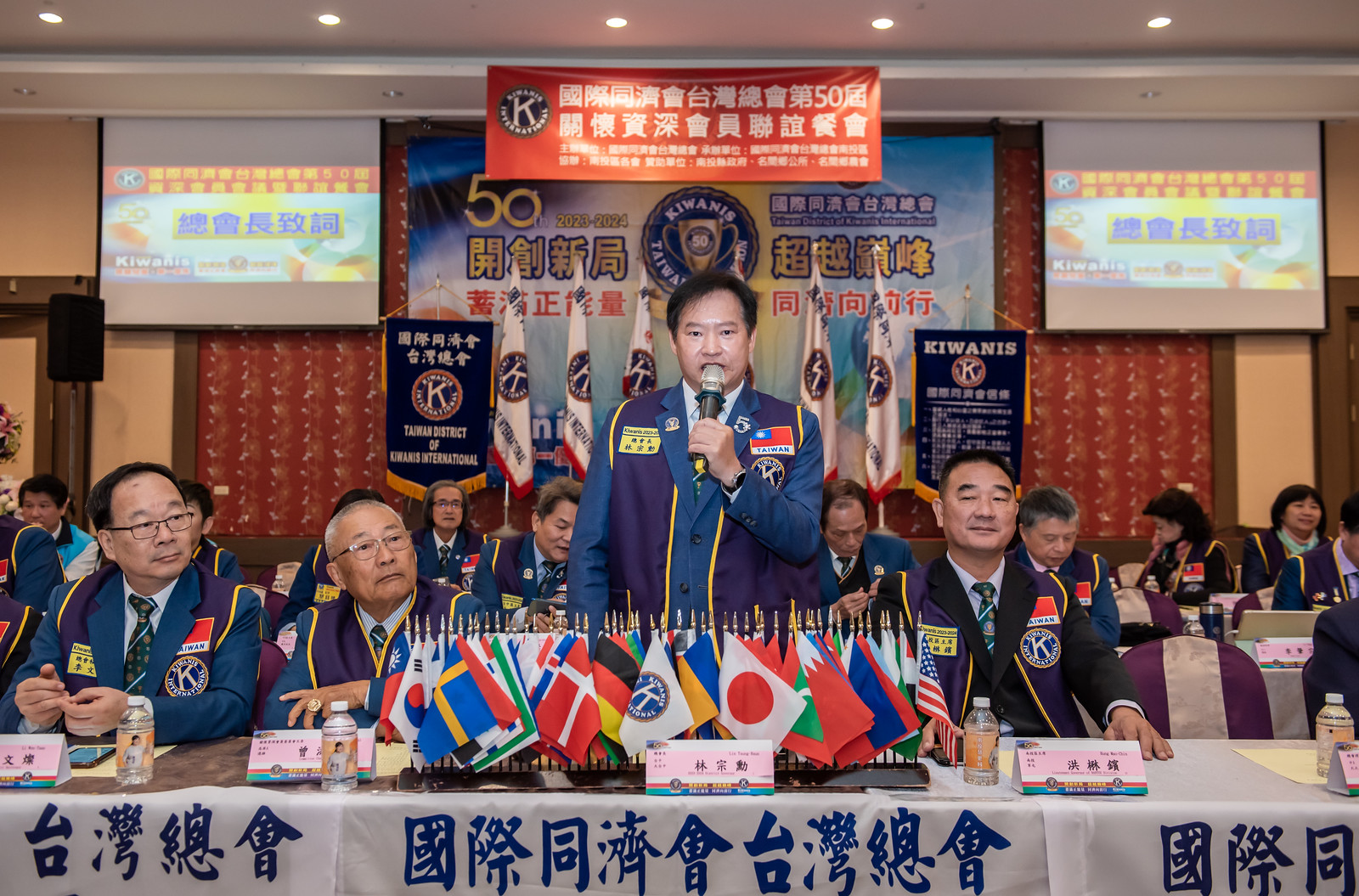In this photograph taken indoors in an elaborate and heavily populated ballroom, an Asian world leader stands authoritatively at the center. The room is arranged for a formal gathering or dinner meeting. The man, in his 40s, has dark hair and is clean-shaven. He is dressed in a purple military-style tunic trimmed in gold over a blue jacket, adorned with badges or military decorations on the lapels. He holds a microphone to his mouth with his left hand, his expression stern and focused as he delivers an important message to the audience. The man's right arm hangs relaxed at his side.

In front of him is a long horizontal table covered with a white cloth bearing blue symbols and upward-pointing arrows. The table is topped with approximately 50 to 60 small international flags, symbolizing a global gathering. Flanking him are several older Asian men; on the left side of the image, two men dressed in similar outfits sit at the table, while on the right side, another elderly man clad in a dark suit with a blue and white patterned tie sits beside an empty chair.

In the background, rows of tables are populated with seated people, all of Asian ethnicity. Suspended from the ceiling are two pull-down screens projecting banners with blue text on light blue backgrounds and red borders at the top. Between the screens hangs a red horizontal banner featuring a logo of a blue circle with a white 'K,' beside which is text in an Asian language. Below this banner, another large screen displays an emblem with a blue shield against a sky-blue background. Surrounding this setup, six white standing flags with blue circles are placed, flanked by vertical blue banners carrying the same logo and more text in an unrecognized Asian script.

The man's intense focus and the ornate setting highlight the significance of the occasion, even though few in the photograph seem to be paying close attention to his address. Nevertheless, his determined demeanor underscores his belief in the importance of his message.